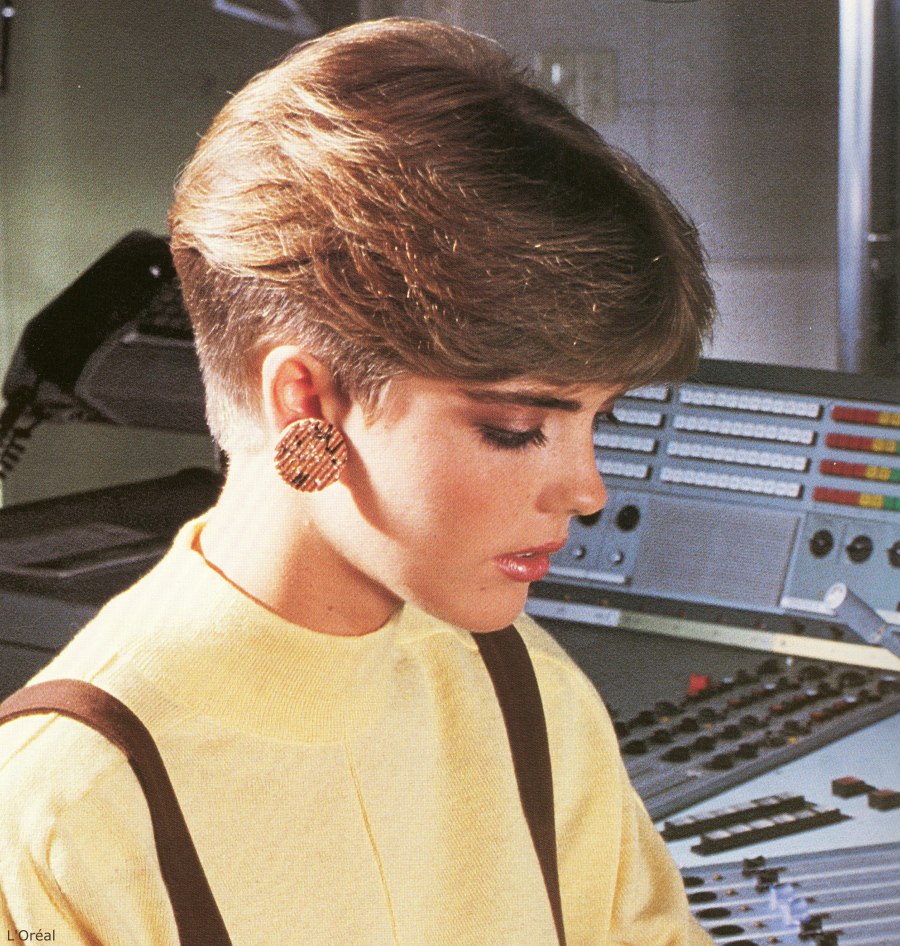The photo depicts a young woman in her early 20s, styled in a distinct 1980s fashion, seated behind an extensive console typical of recording studios or radio stations. Her short pixie haircut is feathered on the sides, almost resembling a tomboyish style that was popular in that era. She wears circular earrings characterized by a design that resembles a Ruffles potato chip with ridged textures and an abstract, Jackson Pollock-style pattern featuring colors mostly in white and black. Her outfit is composed of a yellow, turtleneck-like blouse with brown suspender straps over her shoulders. Her makeup is pronounced, with heavy eye makeup and lipstick, suggesting that she might be posing as a model or in a setting meant for a beauty shot. The background features a light that could be a flashbulb commonly used in photography, adding a professional studio atmosphere. Additionally, there’s a vintage 1980s phone visible, hinting at the time period. At the bottom left corner of the image, the word "L'Oreal" is inscribed, indicating that this photograph might be part of an advertisement for a L'Oreal product.